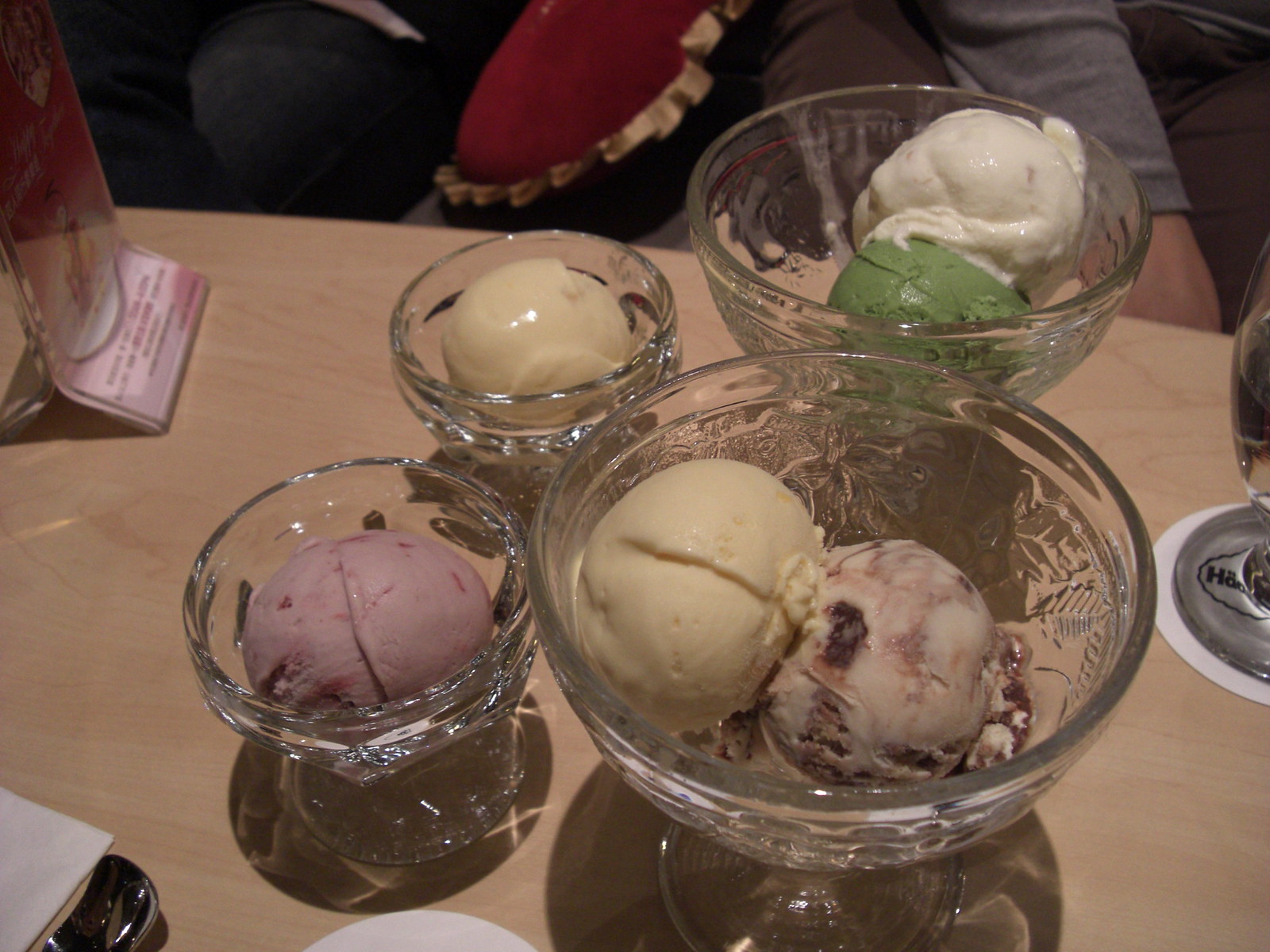The image appears to be taken at a light-wood restaurant table featuring a pink advertisement displayed in a clear plastic holder on the upper left corner. The table is set with four glass bowls of ice cream: the two smaller bowls on the left each containing one scoop - one appears to be caramel and the other a berry flavor. On the right, the two larger bowls each have two scoops of ice cream: a vanilla and mint combination in one, and a caramel and berry in the other. Additionally, a wine glass peeks into the frame from the far right, and a napkin and spoon are partially visible at the bottom left. Though there are people seated, only their arms, feet, and a part of their thighs are visible, along with a red pillow with gold edges on the seat, hinting at a cozy setting.